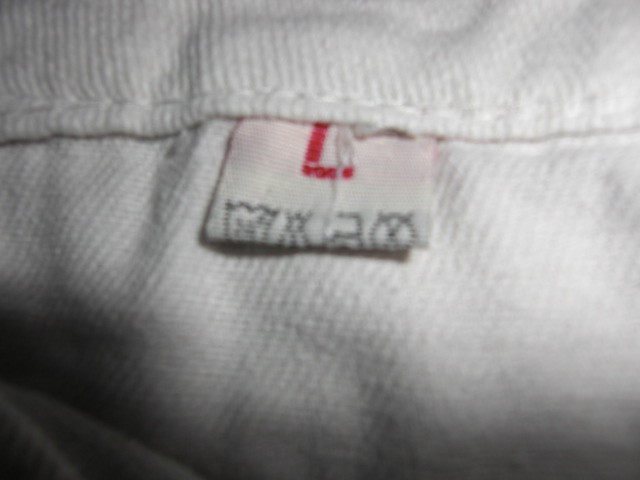This close-up photograph captures a manufacturer tag sewn into the seam of an article of clothing. The image is somewhat blurry and dimly lit, yet it's apparent that the tag is made from bright white material. Prominently displayed on the tag is a large red letter 'L', denoting a size large. Surrounding this letter are various care instruction symbols rendered in gray, though their specific details are hard to discern due to the image's poor clarity. The fabric of the clothing and the tag itself both appear textured, resembling the roughness of white canvas rather than a smooth surface. This textured quality is highlighted despite the overall dark and somewhat unclear presentation of the photograph.